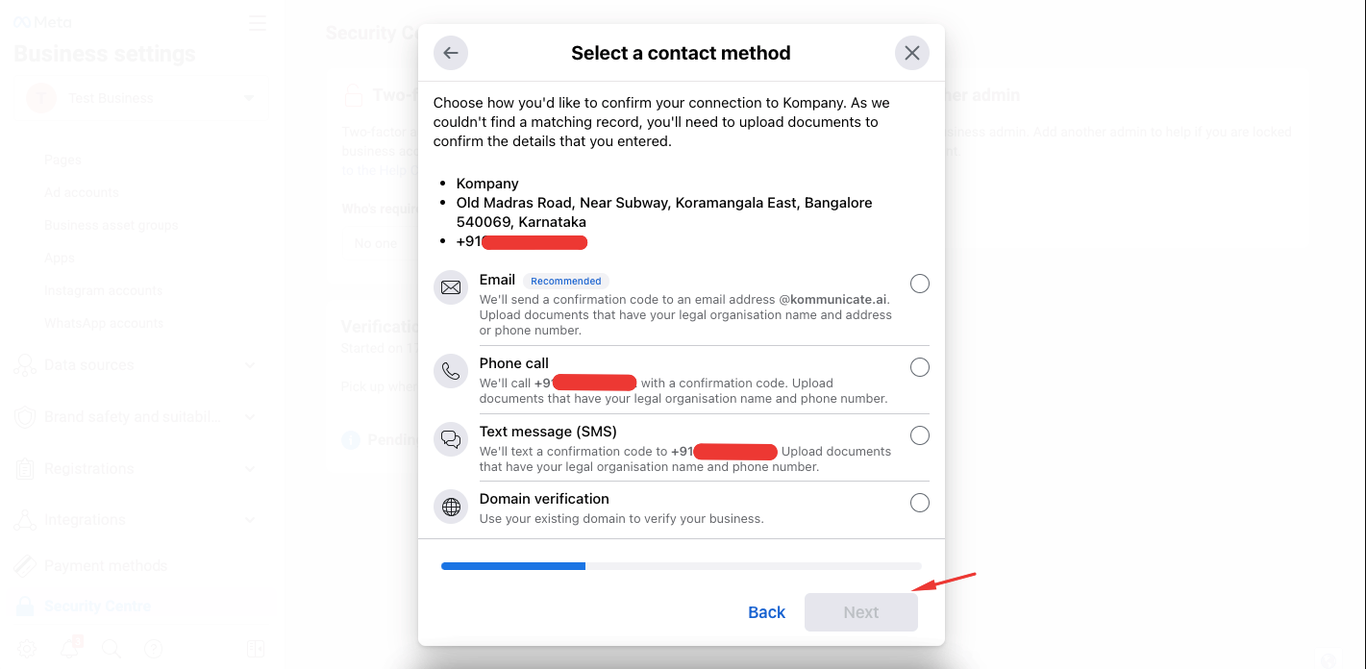In this image, a black-and-white background highlights a user interface prompt titled "Select a Contact Method," displayed in black text at the top. The screen invites users to choose a method for confirming their connection to "Kompany"—notably spelled with a "K"—by uploading documents since no matching records were found. Three bullet points provide further details: the company's name, its address at Old Madras Road near the subway in Koramajanjula East, Bangalore 540069, Karnataka, and a phone number that is strategically obscured by red, curved-edged rectangles for privacy reasons. On the left side of each bullet point, corresponding icons represent contact options: email, phone call, text message (SMS), and domain verification. At the bottom right corner of the image, a red arrow points to the "Next" button, guiding the user to proceed with the process.